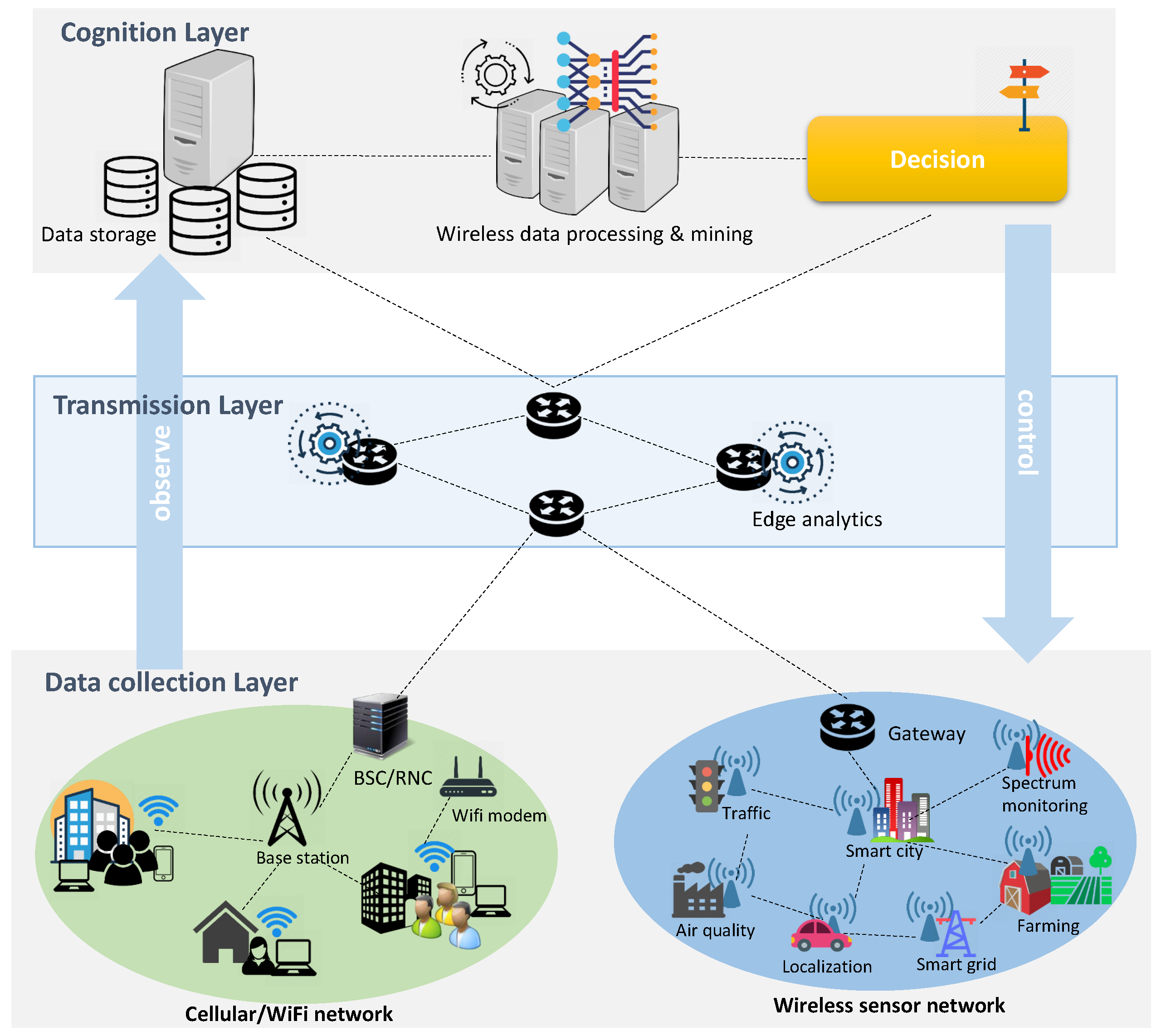This is a detailed diagram likely found in textbooks or educational websites, organized into three distinct layers, each framed within grey and white backgrounds. 

At the very top, labeled as the Cognition Layer, a computer tower is depicted alongside several containers, with the phrase "Cognition Layer Data Storage" clearly indicated. Adjacent to the tower, moving towards the middle, three additional computer towers signify "Wireless Data Processing and Mining." To the right, a prominent yellow rectangle is labeled "Decision."

Descending to the second section called the Transmission Layer, there are multiple black boxes with arrows and gears highlighted in blue, representing "Edge Analytics." Arrows are positioned on both sides; one ascends with the label "Observe," while the other descends marked "Control."

At the bottom, the Data Collection Layer displays two distinct ovals. The left oval, colored green, is identified as the "Cellular Wi-Fi Network," featuring icons such as base stations and Wi-Fi modems. The right blue oval represents the "Wireless Sensor Network" with icons illustrating traffic, gateways, spectrum monitoring, farming, smart grids, localization, air quality, and smart city components. Each component within the ovals helps illustrate the complex network interactions, completing the hierarchical structure of the diagram.